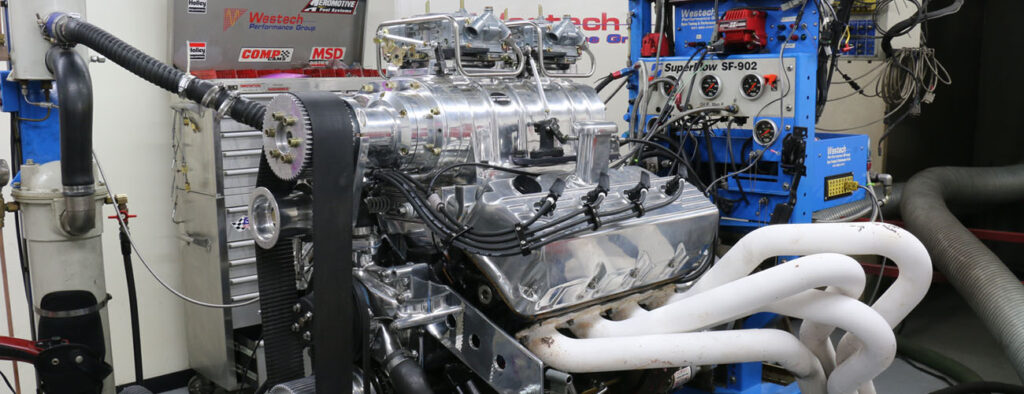This color photograph captures a detailed view of an internal combustion engine positioned in a workshop or factory setting. The engine features a polished silver cover with four visible spark plug wires and large white pipes extending from its bottom. To the left of the engine, a large wheel drive shaft with a black belt is connected to a black hose leading into a gray cylindrical object. Behind the engine stands a large mechanic's toolbox with its top lid open. On the right side of the engine, a blue instrument labeled with "Superflow SF902" and adorned with meters, wires, and hoses, is connected to the engine. This instrument features red switches on top and is accompanied by black text. The background reveals a white wall and the COMP and West Tech logos. The entire scene is a complex assembly of gears, motors, wires, and tubes, creating a chaotic yet clean and organized appearance.